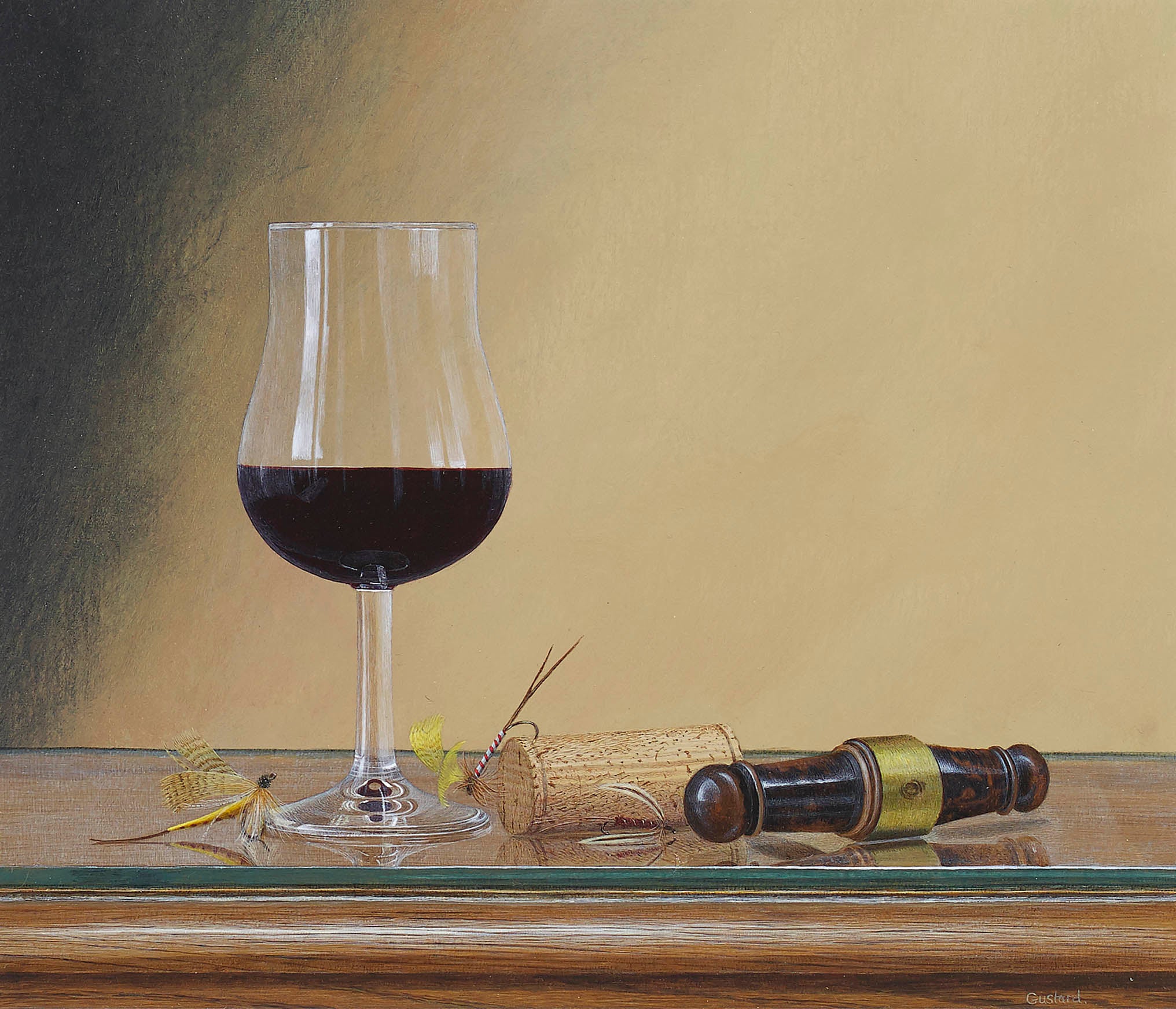The color photograph showcases a crystal wine glass, positioned just left of center on a wooden table. The glass, with a long stem, contains about five ounces of dark red wine. Beneath the glass, there are two fly fishing lures, one resembling a dragonfly with yellow wings. To the right of the wine glass lays a cork, and further right is a wooden bottle opener. The surface appears to be glass-topped wood, with the wooden trim visible in the foreground. The background features a solid color wall, which transitions from darker on the left to lighter around the glass, in shades of brownish beige.